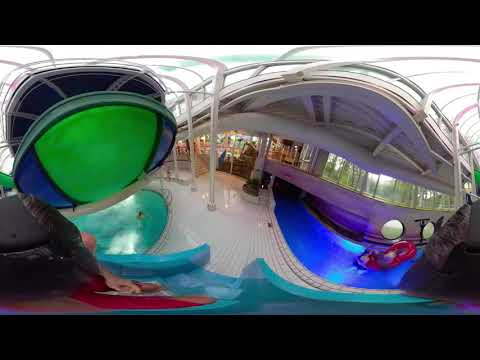The image depicts the interior of a whimsical indoor entertainment area with panoramic distortion, causing the ceiling and floor to appear curved. On the left side of the scene, there's a person partially visible, sliding into a turquoise pool of water, which features little handles for exiting the pool. Above this pool, a green spherical structure encased in a blue container or holder hangs from the ceiling, casting an intriguing glow over the area. Further to the right, another pool of bright blue water is visible, with someone or some object—potentially a bumper boat—floating inside. Adjacent to this is a dark blue water slide that appears to have a red raft with a person in it. Between the pools, there's a tiled floor with supporting pillars that extend up toward a glass ceiling. To the far right, there's a stream or blue track with a red car riding on it, and towards the background, a walkway with pillars supporting a covered beam structure can be seen. The overall effect is a vibrant, multi-leveled play area possibly located within a mall or pavilion, with various water activities and structures adding to the festive atmosphere.